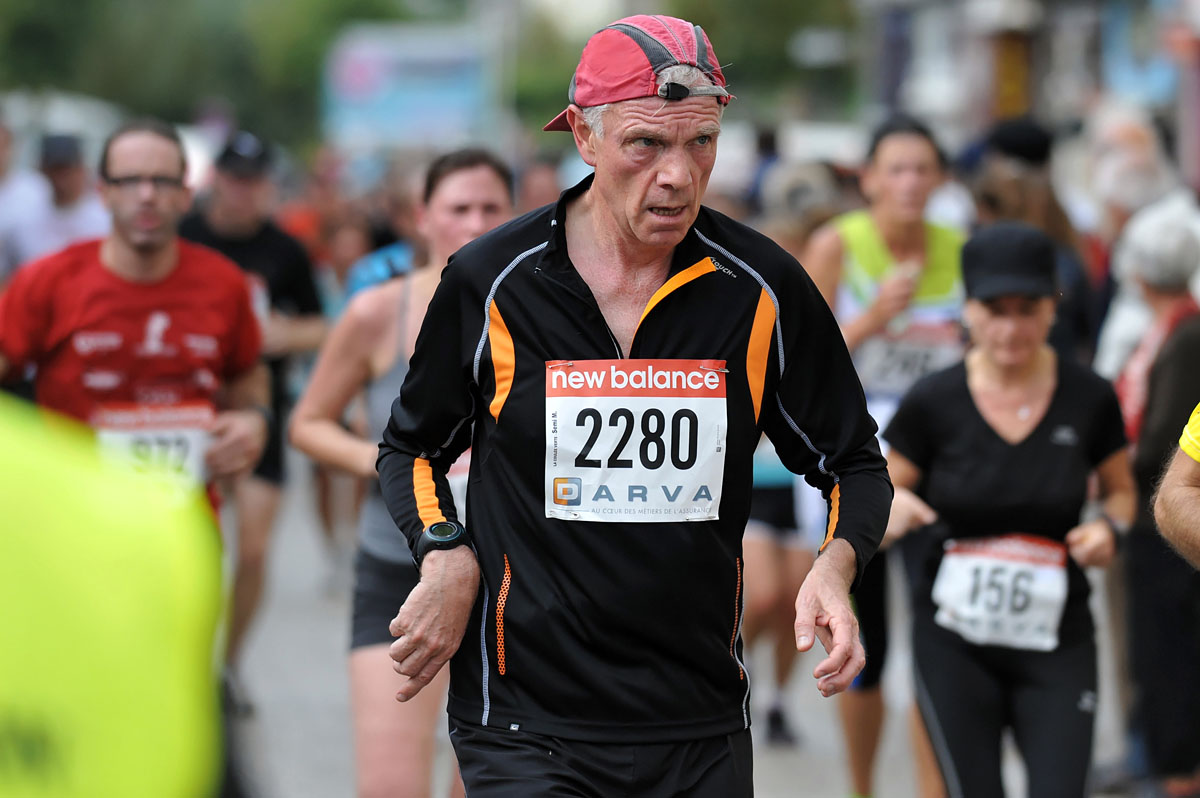This detailed photograph captures a marathon scene, with a diverse group of men and women running together outdoors during the daytime. Central to the image is a prominent older man wearing a lightweight black jacket adorned with orange and gray accents. His jacket displays a New Balance tag with the number "2280" and a possible sponsor name that appears to be "Arva." The man also sports a pink or possibly red cap worn backward over his gray hair and a black watch on his right wrist. In his immediate surroundings are other participants, such as a man in a red shirt with the number "972" and a woman in a gray tank top and black shorts. Another female runner is clad in black pants and a shirt, with the number "156" visible on her tag, paired with a black hat. An additional participant stands out in a lime green or yellow and white tank top. The background of the image gradually blurs, featuring more indistinct runners and some trees, suggesting motion and depth in the scene.